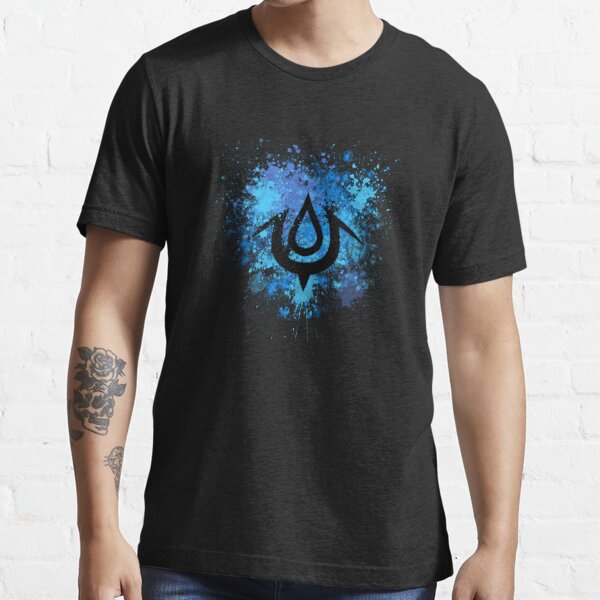This photograph features a male model standing against a backdrop of white bricks. The focus is on his attire and his upper body, specifically the area from his neck to his waist. He is wearing a black half-sleeve t-shirt adorned with a striking design on the chest. The design consists of blue splashes framing a central black symbol, which resembles a teardrop with a curved, pointed arch below it. The model's left arm is visible, showcasing tattoos including a detailed skull with a rose growing out of it, and hints of additional floral and leaf patterns. Part of his blue jeans is also faintly visible. The overall composition suggests that the primary purpose of this image is to highlight and advertise the t-shirt he is wearing.